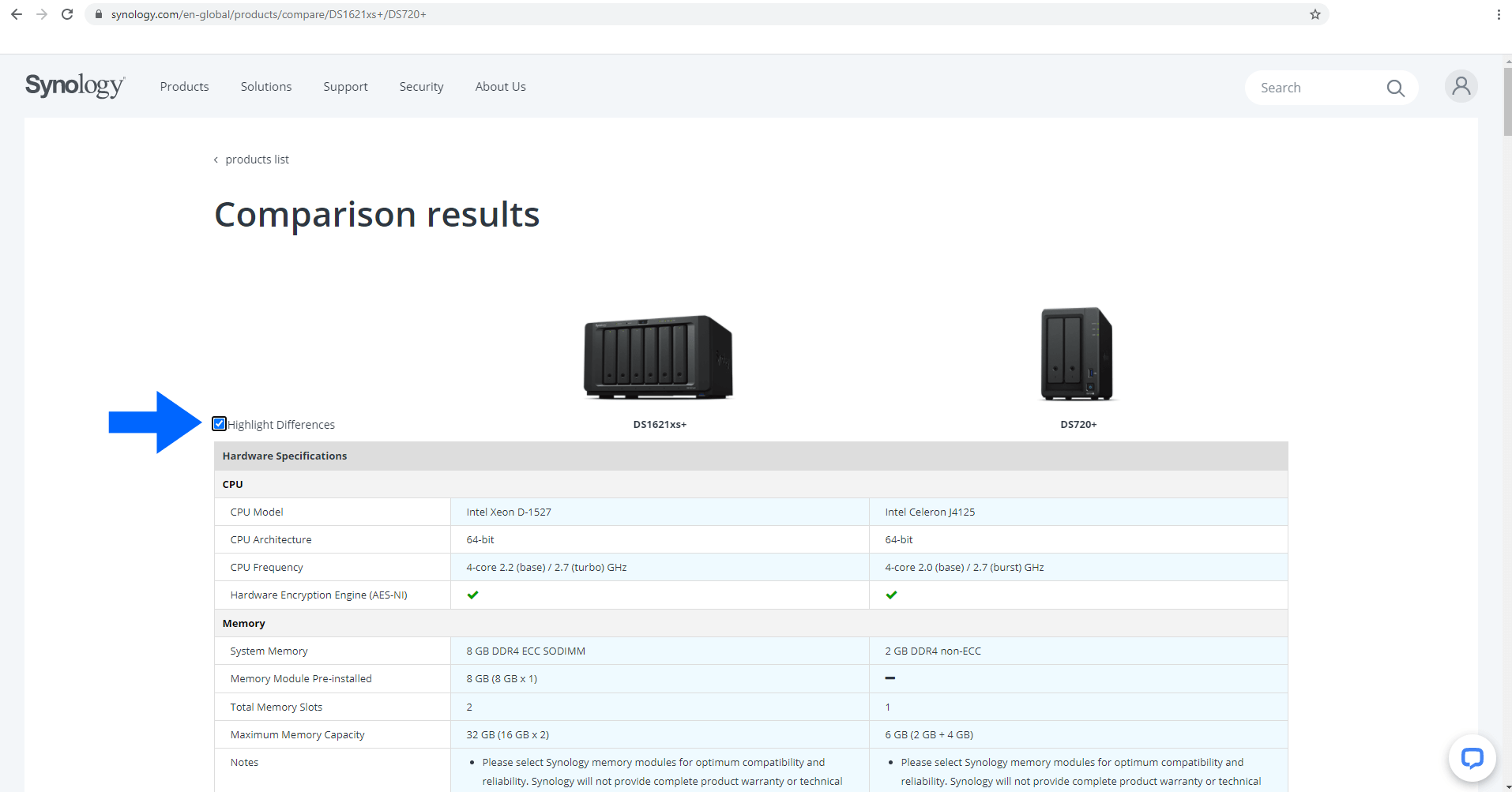This screenshot captures a webpage from Synology.com. At the very top, there is a search bar displaying "Synology.com" and the rest of the website URL. The page prominently features the Synology logo in black, followed by navigation options: Products, Solutions, Support, Security, and About Us.

Dominating the center of the page is a large white box with the title "Product List" in bold black letters, followed by the subtitle "Comparison Results." Below this section are images of two black Synology devices, positioned side by side. A blue arrow on the left side of the page points towards a box labeled "Highlight Differences," aimed at aiding users in comparing the two products.

The page then delves into detailed product information, starting with "Hardware Specifications." Under this section, various specifications are listed, each preceded by a title in black: CPU, Memory, and others. The CPU section includes specifications like CPU Model, CPU Architecture, CPU Frequency, and Hardware Encryption Engine, with corresponding options listed. Similarly, the Memory section provides options for System Memory, Memory Module Pre-installed, Total Memory Slots, Maximum Memory Capacity, and Notes.

The information is presented in rectangular bars that vary in color, predominantly white, gray, or blue, ensuring that details are clear and organized for user convenience.